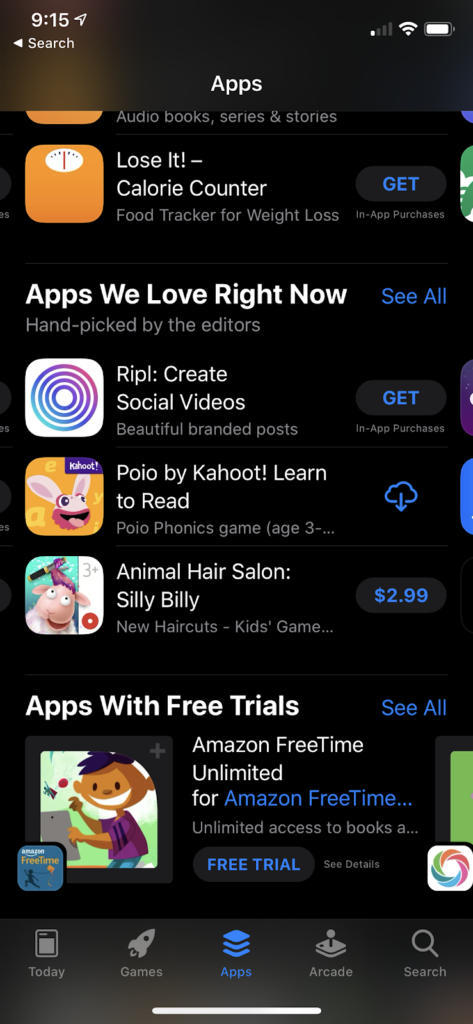This screenshot displays a typical smartphone screen with a predominantly black background. 

At the top of the screen, on the left-hand side, the time is shown as 9:15, accompanied by a right-pointing arrow. Just below this, there is a search bar with a left-pointing arrow. On the top right corner, the signal strength is indicated by two small bars, suggesting weak cellular service, while the Wi-Fi signal is strong and the battery is fully charged. 

Below these, the user has a collection of app icons. The first icon is partially cut off but appears to relate to audiobooks, series, and stories. Directly beneath this, there is an orange icon resembling a scale, labeled "Lose It!"—a calorie counter and food tracker for weight loss, with an option to "Get" the app. 

Continuing downward, a section titled "Apps We Love Right Now" can be seen, suggesting these are editor's picks. The first app in this section features a blue disc on a white background and is named "RIPL," used for creating social videos and beautifully branded posts, available for download with a "Get" button. Next to it, there's an app with an icon of a big-mouthed rabbit on an orange background, titled "POJO by Kahoot! Learn to Read" with a POJO Phonics Game suitable for ages 3+, indicated by a cloud download icon. Another highlighted app shows a pig getting a haircut, titled "Animal Hair Salon: Silly Billy New Haircuts," which is a kids' game priced at $2.99.

Lastly, there is a section called "Apps with Free Trials," featuring "Amazon FreeTime Unlimited," which offers access to books with a free trial option.